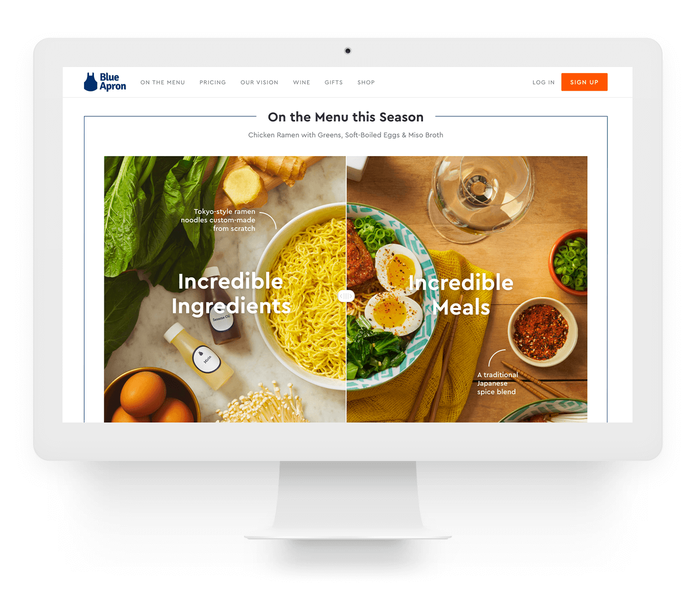In this detailed image, a light gray computer forms the backdrop, featuring a small dot at the top center, which is the camera lens. In the foreground, there is a prominent white box. In the upper left corner of this box, the Blue Apron logo is displayed in blue, accompanied by an illustration of a blue apron. The top navigation bar includes menu options like "On the Menu," "Pricing," "Our Vision," "Wine," "Gifts," and "Shop." On the right side of the navigation bar, there is a "Log In" link and a prominent red "Sign Up" button.

Below this, a thin blue line demarcates another white box with a blue border. This section highlights seasonal menu items, specifically "Chicken Ramen with Greens and Soft-Boiled Eggs" and "Miso Borscht." Accompanying this text is an illustrative image divided into two sides. One side showcases vibrant ingredients under the heading "Incredible Ingredients," including various spices. The other side, labeled "Incredible Meals," presents a bowl of meticulously arranged food. The bowl features noodles on one side, and greens, tomatoes, and halved soft-boiled eggs on the other.